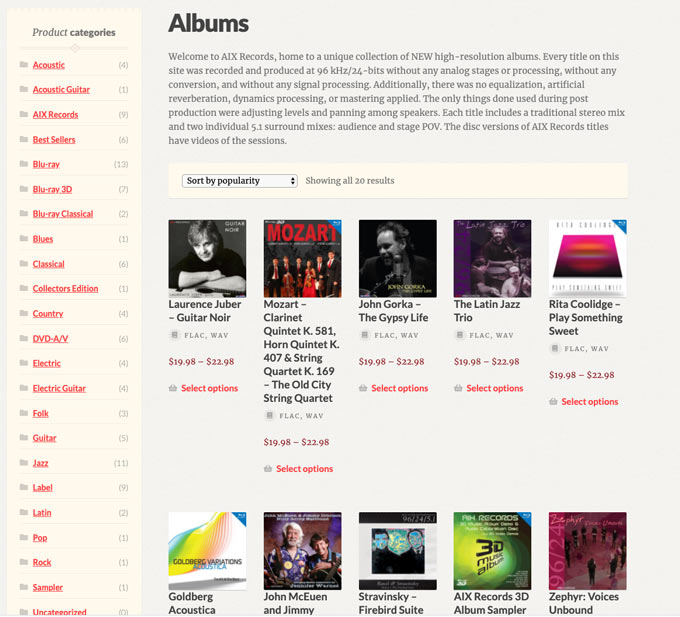The image depicts the homepage of AIX Records, a site renowned for its unique collection of high-resolution albums. The homepage prominently features a selection of ten album covers, sorted by popularity, offered as illustrative examples. Among the featured albums are "Guitar Noir" by Lawrence Duber, "The Latin Jazz Trio," and "Play Something Sweet" by Rita Coolidge. These albums are available for purchase in high-quality FLAC or WAV file formats, with prices ranging from $19.98 to $22.98. AIX Records takes pride in the fact that every title available on the site was meticulously recorded and produced at 96kHz and 24 bits, without the use of any analog stages, conversions, or signal processing, ensuring a pure and high-fidelity listening experience.